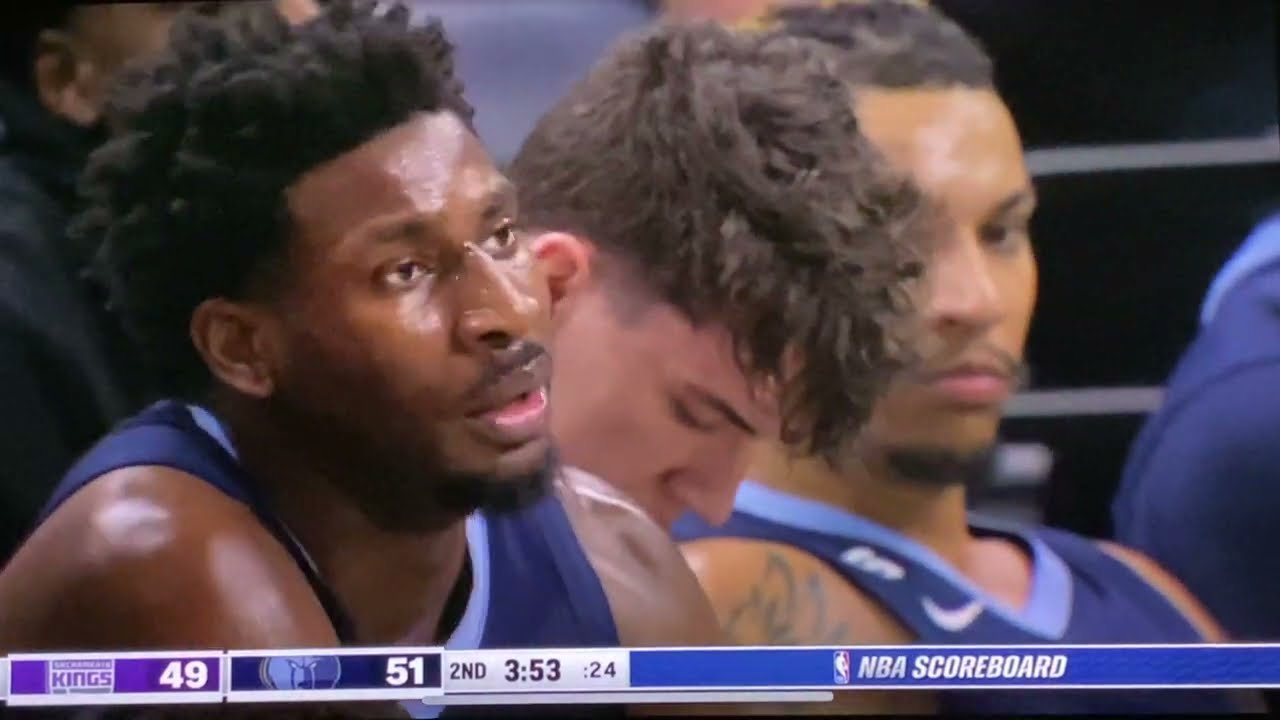The image is a close-up shot of three dejected basketball players sitting on the bench during a game, as captured from a TV broadcast. The player on the left is a dark-skinned African American man with wild dark brown hair and a pronounced nose, his mouth slightly open, showing signs of sweat on his face and shoulders. He wears a navy blue jersey with light blue trim, featuring the Nike swoosh logo on the left. The player in the center is a white male with dark hair, his flushed red face looking down in disappointment. To his right is a partially obscured Hispanic man with dark hair, a dark mustache, and a bit of a beard, also in a navy blue jersey. The scoreboard at the bottom of the screen shows the Kings in purple with 49 points, against another team with a wolf emblem, which has 51 points. The game is in the second quarter with 3 minutes and 53 seconds remaining. The NBA scoreboard is displayed in white font against a blue background.